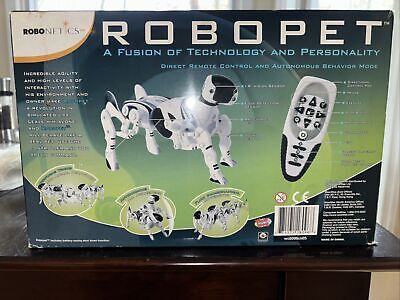This is a photograph of the box for the Robopet, a futuristic robotic pet. The product name "Robopet" is prominently displayed at the top in a font similar to that used in Terminator, conveying a high-tech aesthetic. Below the name, in white and blue fonts, is the slogan "A fusion of technology and personality." The front cover features an image of the Robopet, a four-legged robotic dog predominantly white with black accents, especially noticeable around its head with a black plate instead of an actual face. Additional images show the pet in various poses, displayed within circular frames against a green gradient background. Also featured is an image of the remote control, which is white with black buttons and accents, shaped like an ice cream cone with eight primary buttons, a power button, and three elongated buttons. The box is placed on a polished dark wooden table, reminiscent of redwood, and is set against a backdrop of a window with vertical blinds, allowing light to filter through.